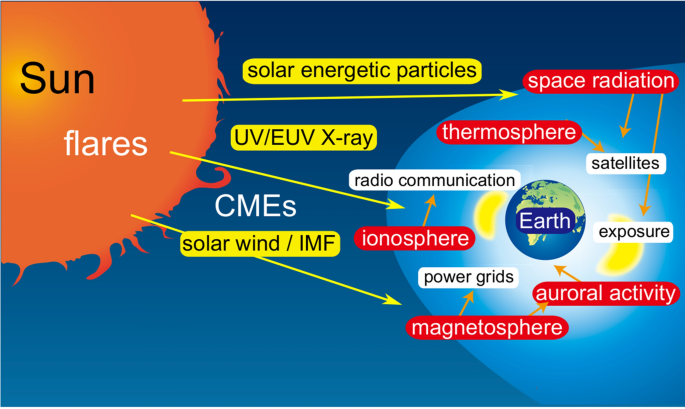This vibrant, detailed diagram illustrates the effects of the Sun on Earth and appears to be sourced from a PowerPoint slide or textbook. The image features a blue background with a stylized, digitally drawn Sun on the left. The Sun, depicted in bright orange, displays the label "sun" in black text with "flares" underneath in white. From the Sun, three yellow arrows extend towards Earth, each annotated with different solar phenomena. The first arrow represents "solar energetic particles," the second indicates "UV/EUV X-ray," and the third depicts "solar wind/IMF." 

Midway between the Sun and the Earth, "CMEs" is prominently displayed in capital letters. The Earth itself, rendered as a green and blue cartoon-like digital image, sits on the right side of the diagram. Surrounding the Earth are several red circular boxes labeled "space radiation," "thermosphere," "ionosphere," "auroral activity," and "magnetosphere," each with orange arrows connecting them to the white boxes.

These white boxes denote the impacts on various Earth systems, labeled as "radio communication," "satellites," "exposure," and "power grids." Specifically, arrows trace from "space radiation" to "satellites" and "exposure," from "thermosphere" to "satellites," from "ionosphere" to "radio communication," and from "magnetosphere" to "power grids." This intricate diagram visually explains how solar activities like solar flares and energetic particles propel through space to influence Earth's technologies and atmospheric layers.